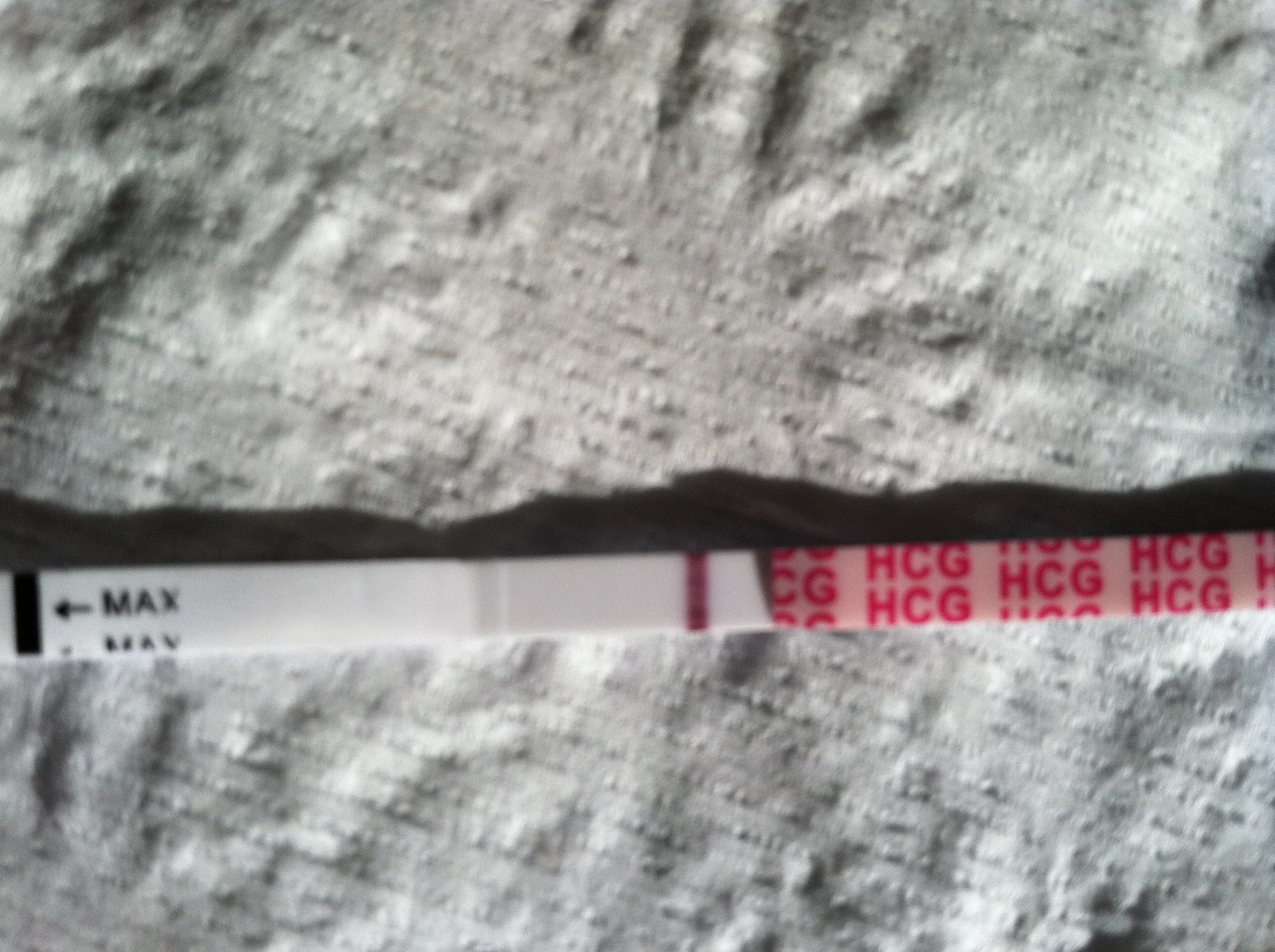This close-up image captures two pieces of stone, likely tiles, positioned one on top of the other. The bottom stone has a flat, smooth top edge, indicative of having been precisely cut. In contrast, the top stone exhibits a rough, jagged bottom edge, suggesting it has recently been broken or is yet to be smoothed out. Sandwiched between the stones is a strip of tape. The left side of this tape is predominantly white, featuring black lettering that reads "MAX" alongside a black arrow pointing to the left. The right side of the tape is covered with a transparent film adorned with rows of red "HCG" text, repeating from top to bottom and left to right. The setup suggests that the tape is potentially being used as a guide or marker, perhaps in the process of cutting or aligning these stones for use in constructing a wall or a floor. The detail and alignment imply a meticulous approach to ensuring these stones fit together seamlessly.